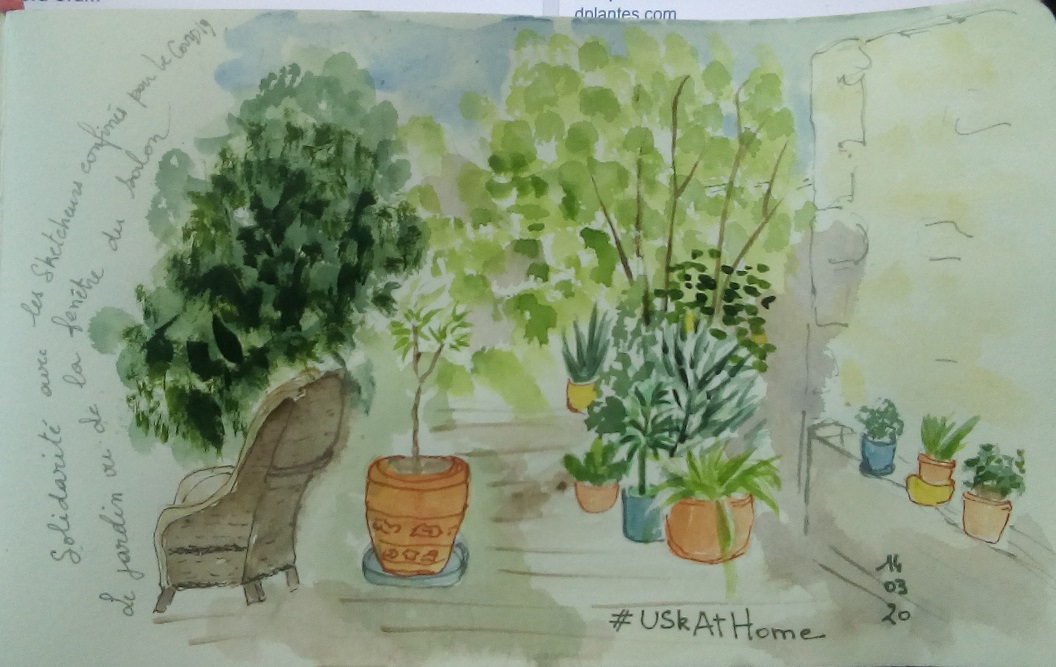This watercolor-style painting depicts a cozy patio scene. The ground is illustrated with line work and features a spotty brown coloration, representing a wooden deck. A yellowish wall serves as the backdrop, adding warmth to the composition. Brown and blue planters, filled with lush green foliage, are scattered around, adding pops of color and life. A prominent orange pot, resting in a blue saucer, holds a budding seedling tree, signifying growth and new beginnings. Additional orange and blue planters, each containing various styles of green plants, provide a diverse array of greenery. In the background, light green trees on the right and dark green trees on the left frame the scene, enhancing the natural ambiance. A charming brown wicker chair is positioned to the left, inviting relaxation. At the bottom of the painting, the caption reads "#USK at Home," suggesting it is part of the Urban Sketchers community.